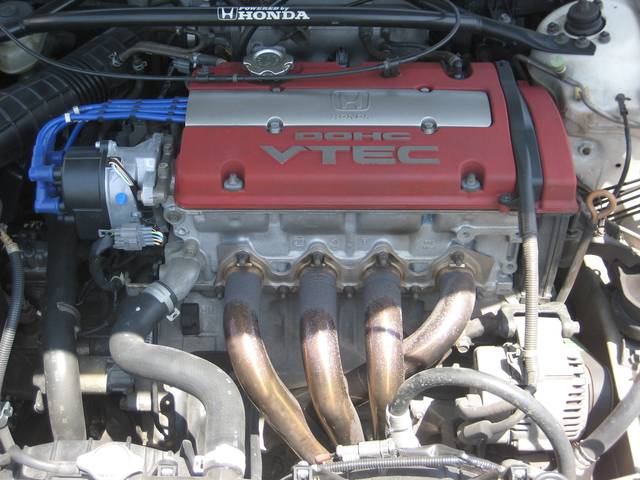This is a detailed color photograph showcasing the engine compartment of a vehicle, specifically highlighting a Honda engine. At the very top of the image, the roof of the vehicle is visible. Prominently displayed in the center, in white letters, is the Honda insignia accompanied by the phrase "powered by Honda." Below this, the engine's red cover is clearly visible, which is marked with "DOHC" and "VTEC" in grey lettering. The cover features a brushed aluminum strip running down the center, secured by four nuts at each corner. On the left side, bright blue spark plug wires can be seen emerging from this strip. Additionally, there is a collection of gold and silver-toned tubes and black hoses in the lower part of the engine, with sunlight casting highlights upon them. The photograph captures a detailed and illuminated view of the engine components, with a greyish sky peeking through a window in the upper right corner, adding an atmospheric touch to the technical display.